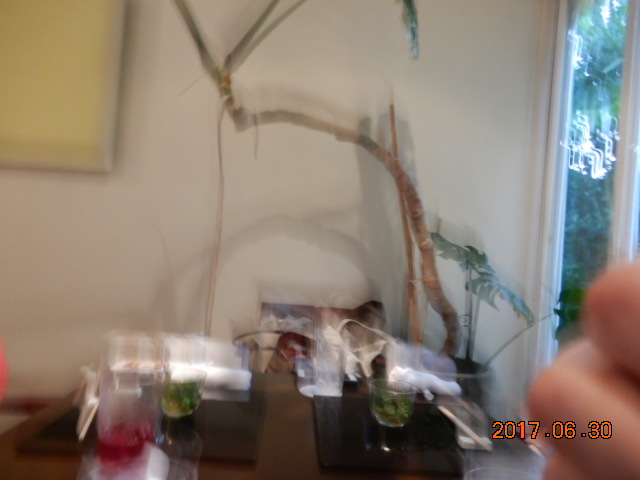This slightly blurry photo, dated June 30th, 2017, captures a corner of a room in a private residence. The setting includes an off-white wall and a window or possibly a glass door with a white frame. In the upper left-hand corner hangs a yellow painting, adding a splash of color to the scene. Dominating the corner is a large indoor plant in a substantial pot, featuring a brown, bent trunk with a few leaves at the bottom.

On a cluttered brown tabletop below, several personal items are visible despite some blurriness. There is a short glass and a pitcher containing a pink liquid. A few folded washcloths or possibly white paper towels are also present. A small glass container with unidentified greenery and another small potted plant with dark soil are near these objects. Adding a human element, the bent fingers of an unseen person emerge along the right edge of the frame. The overall scene is an intimate snapshot of a lived-in, thoughtfully decorated space.